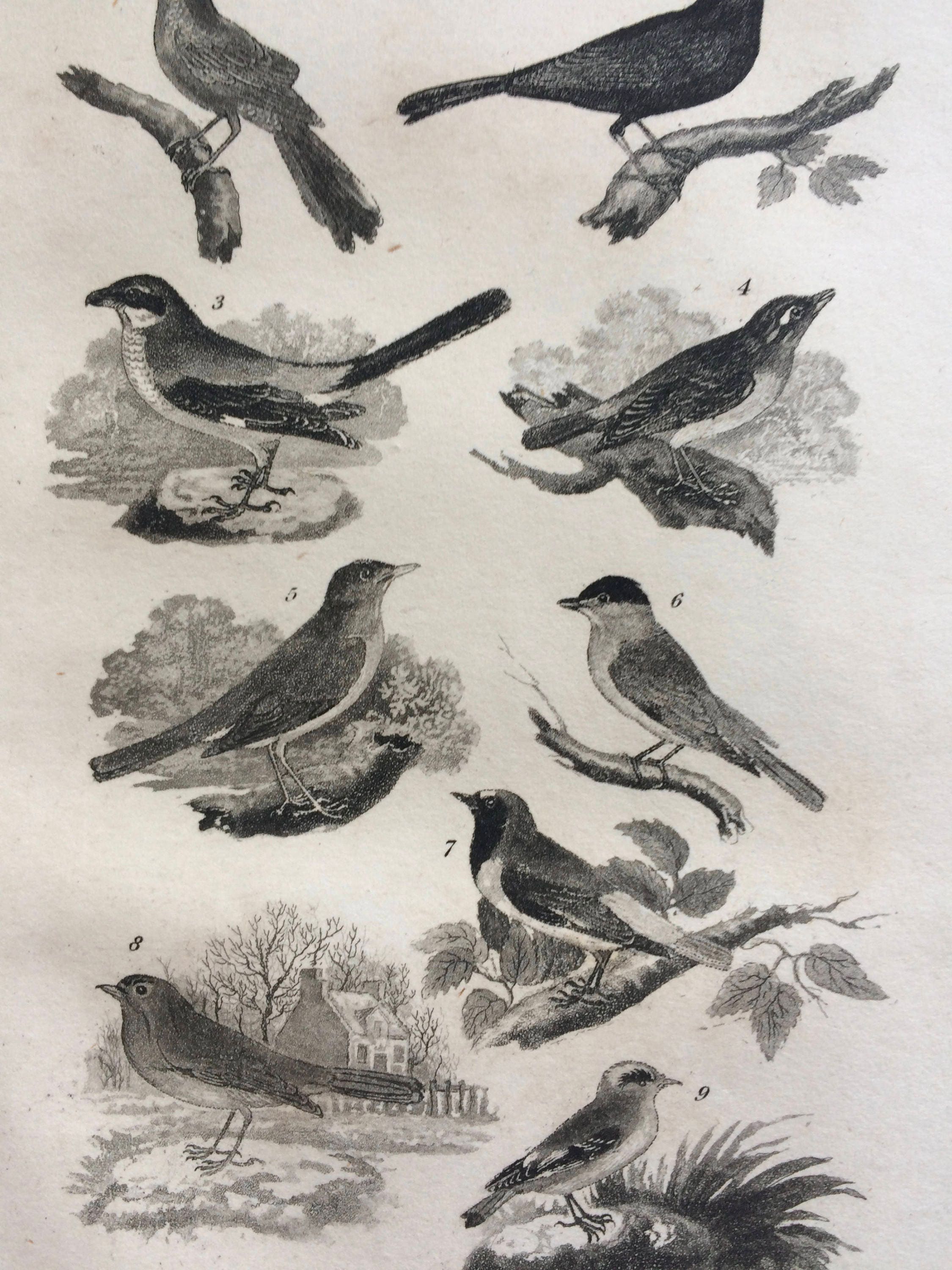The image displays a series of nine detailed black and white illustrations of small birds, each labeled and numbered from 3 to 9, with the top two birds (presumably 1 and 2) partially cropped out so you can't see their heads. These birds are arranged with four on each side, and one at the bottom center, creating a symmetric layout. The illustrations depict the birds either perched on tree branches or stones, and one image includes a bird with a background of a house and a tree, adding a touch of context. Each bird is intricately drawn in dark gray pencil against an off-white, almost gray, background. The birds vary slightly in appearance, resembling different species of sparrows, with minor variations in head color and tail length, giving each bird a unique yet cohesive aesthetic.